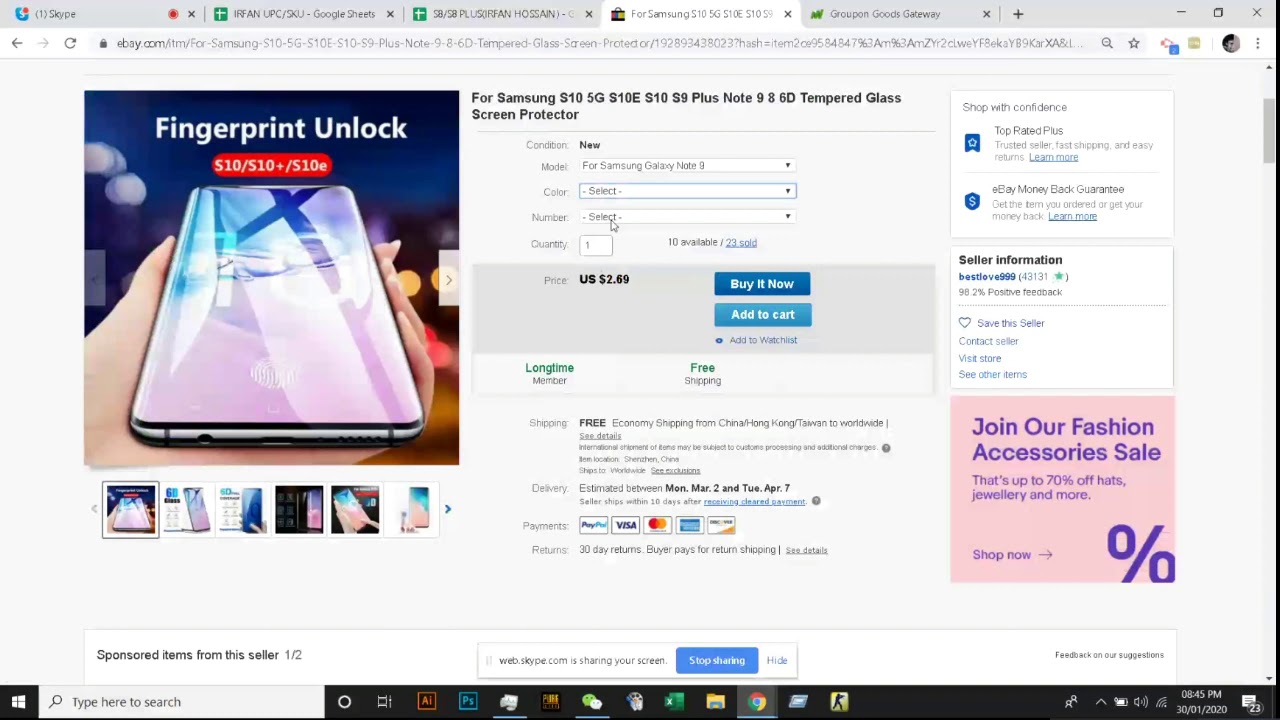The image is a screenshot captured from a Windows computer, specifically while using the Google Chrome web browser. The focus of the screenshot is on an eBay product listing for a fingerprint unlock tempered glass screen protector, compatible with various Samsung models including the S10 5G, S10e, S10, S9+, Note 9, and Note 8. The listing is clearly identified on eBay, evidenced by the interface and the personal knowledge of the original narrator. The page's background displays a basic beige color commonly seen on eBay's platform.

To the right of the main content, there is an advertisement, suggesting the user is indeed browsing through Google Chrome. Multiple tabs are open in the browser, although the exact details of all tabs are not clear. One of the visible tabs features a green and white cross, potentially related to a Samsung-related site or application. Another tab is dedicated to the eBay listing being described.

The user is logged into their Google account in Chrome, indicated by a user-uploaded picture visible at the top of the browser, next to the Chrome settings menu represented by three vertical bars. The screenshot captures a scene where someone is navigating through an online shopping session, poised to purchase a screen protector for their Samsung device on a Windows 10 or 11 computer.